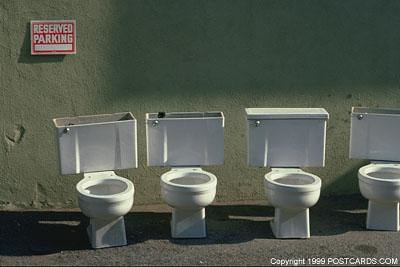The image features a light green concrete wall adorned with a reserved parking sign in the top left corner. The sign has a red background with white lettering that reads "Reserved Parking," and below the text is a bold, horizontal white line. In the bottom right corner of the sign, there is small white text that says "© 1999 postcards.com". Positioned against the wall are four white porcelain toilet bowls arranged in a row. The third toilet from the left is the only one with a tank lid, while the other three are without. None of the toilets have seats, and they are unconnected to any plumbing, sitting directly on gravel. The scene appears to be outdoors, captured likely during the day as the toilets cast distinct shadows. The wall itself has visible chunks missing from the surface, adding a rough texture to the backdrop.